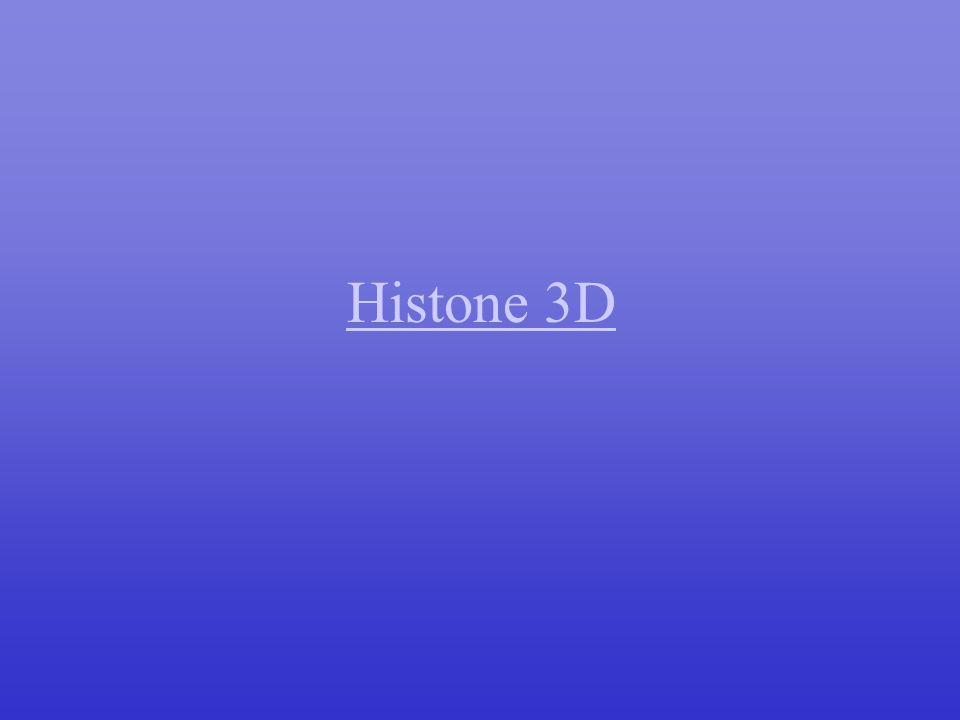The image is a simple blue square graphic featuring a gradient background that transitions from a dark blue at the bottom to a lighter blue at the top. At the center of the image, the words "Histone 3D" are prominently displayed in white serif font, with a capital "H" in "Histone" and a capital "D" in "3D." The phrase "Histone 3D" is underlined with a thin white line extending from the start of "Histone" to the end of "3D." The overall simplicity and clear emphasis on the text likely serve as an effective advertising tactic, making the phrase memorable even if viewers are unfamiliar with its meaning.